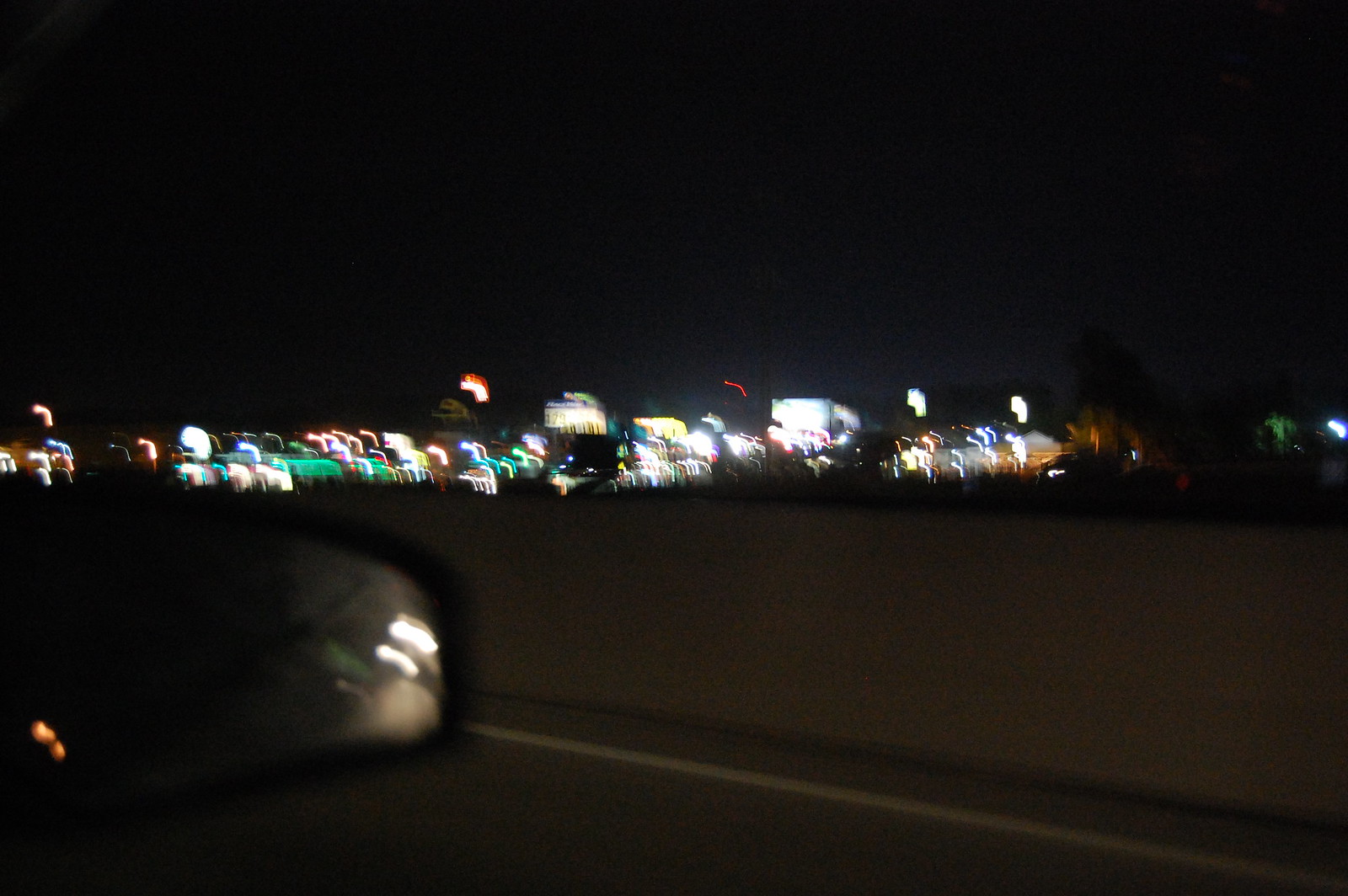The image is a blurry, rectangular photograph taken at night from the passenger side window of a moving car. The road visible in the photo features a dark gray asphalt with a white line along the edge and a small concrete barrier. In the bottom left corner, the car's trapezoidal-shaped side mirror slightly reflects the streetlights behind. In the far distance, the blurry lights of a large city illuminate the darkness, suggesting an urban area with at least 20 buildings, potentially reminiscent of a vibrant downtown, possibly even akin to Las Vegas. The buildings are adorned with diverse colored lights, including white, orange, green, clear, and red hues. To the right, some tall trees stand in contrast against the pitch-black sky. Everything in the picture appears distorted and in motion, contributing to the overall abstract and dynamic feel of the nighttime cityscape captured from a moving vehicle.